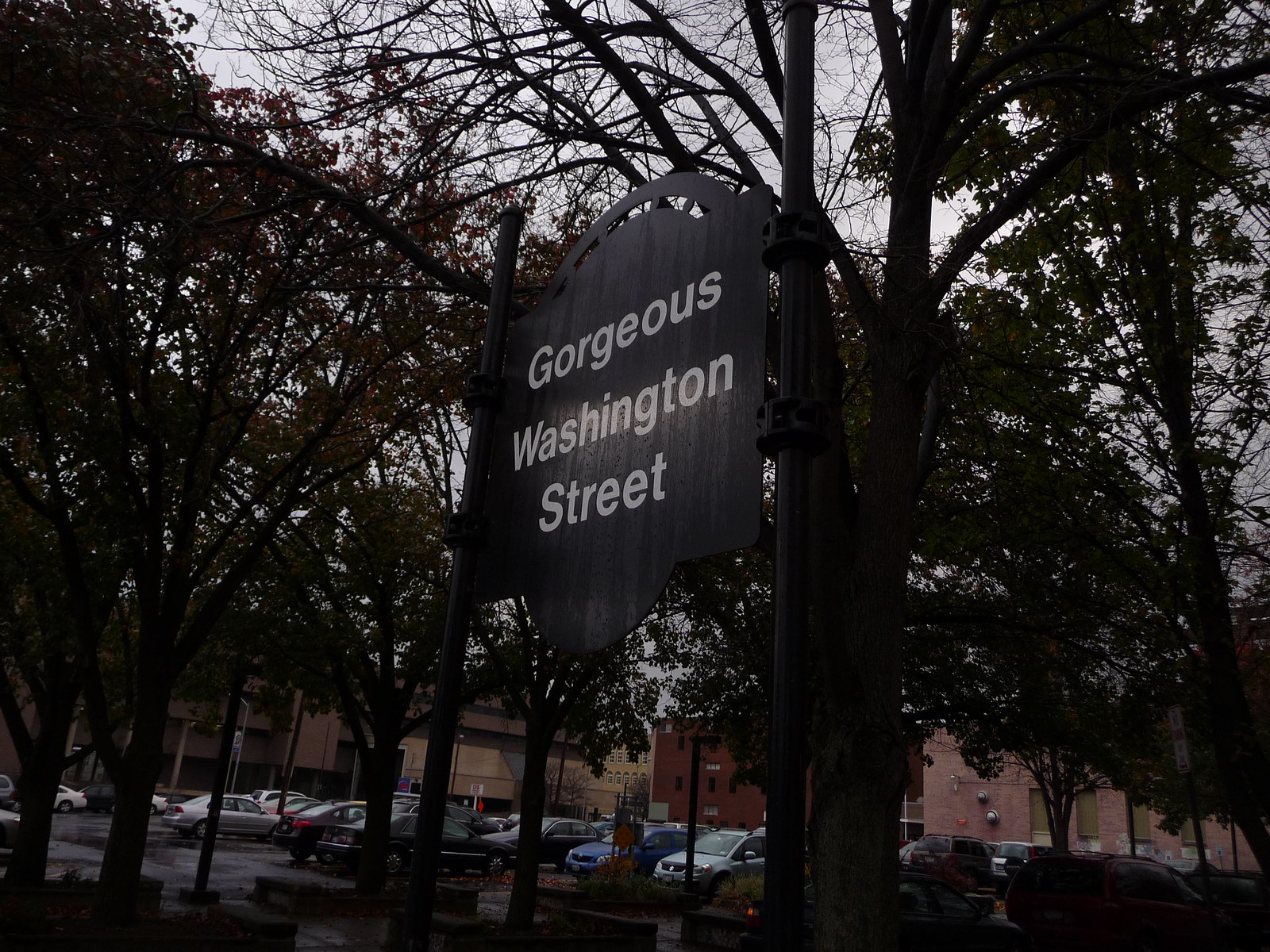This color image combines elements of both realism and surrealism, creating a striking, somewhat disorienting visual effect. The bottom fifth or quarter of the image is in full color, featuring a range of buildings with red and brown walls. A line of cars, including a distinctly blue one and several grey ones, are also colored in this area. The upper portion of the image, however, transitions to black and white. Silhouetted tree shadows, some with leaves and some bare, reach up toward a greyish-white sky, enhancing the eerie atmosphere. At the center of the image, a black, almost hexagonal or possibly star-shaped sign stands out, bearing the text "gorgeous Washington Street" in greyish (or possibly white) lettering, illuminated by a subtle hint of light. The overall effect of the image feels both strange and artificial, leading one to question whether it was generated by AI or manipulated with an unusual filter.